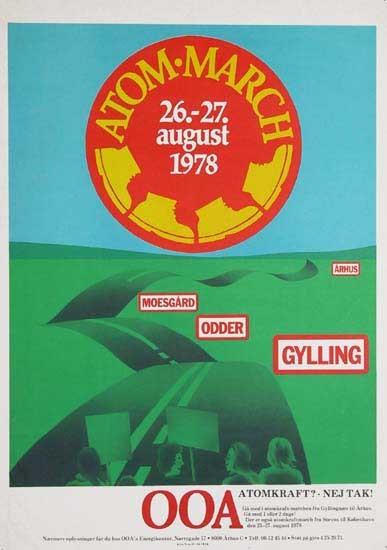The image is a detailed poster featuring a road winding through artistically depicted green hills under a blue sky. At the bottom, a group of people in green and black are holding picket signs, suggesting a protest. The top of the poster showcases a prominent red circle with the yellow text "Atom March." Below, in white letters, it reads "26-27 August 1978." Further down, four yellow shoes are arranged in a counterclockwise format. On the green field, several red-bordered squares contain various words like "Gilling," "Otter," "Moesgaard," and "Mollusc." A white border at the bottom features red text, "OOA," and additional words including "Atomcraft Nishtok." The imagery and text together appear to promote an event or cause, accentuated by its vivid colors and structured layout.